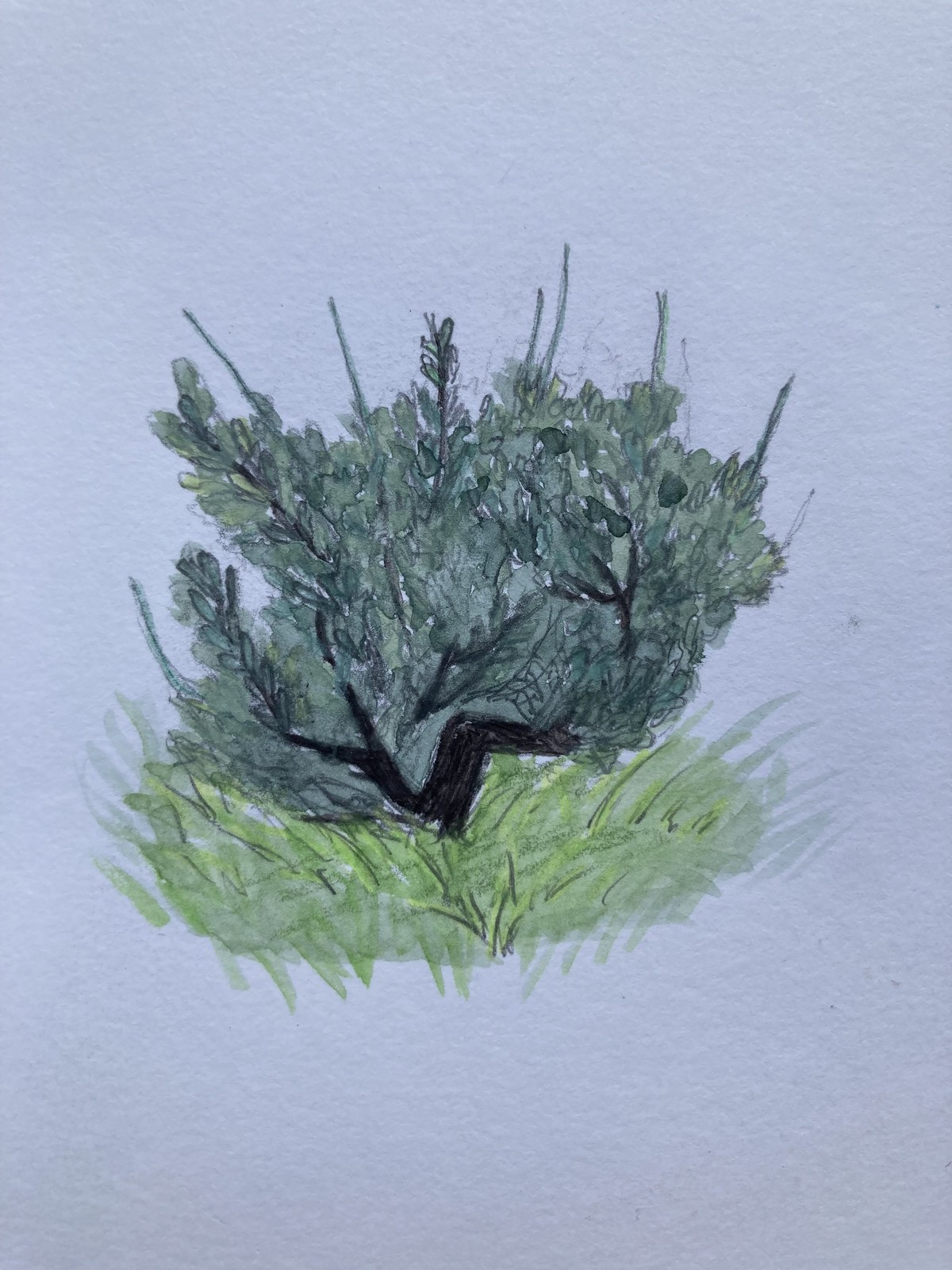The image showcases a photograph of a pencil and watercolor drawing on light or white paper. Central to the composition is an intricately detailed tree, characterized by a combination of mediums: watercolor paints and colored pencils. The base of the drawing features a patch of grass, rendered in varying shades of light and dark green which illustrate the texture and individual blades of grass. Ascending from this grassy foundation is the tree, whose trunk and branches are shaded in dark brown and black, creating a sense of depth and structure. The branches extend horizontally to both the left and right, adorned with dark green leaves arranged in small clusters as well as some random protruding sticks. The background of the drawing remains a plain light gray, helping to accentuate the tree and grass in the foreground. Overall, the drawing captures a realistic and textured depiction of a tree on a grassy patch from a frontal viewpoint.